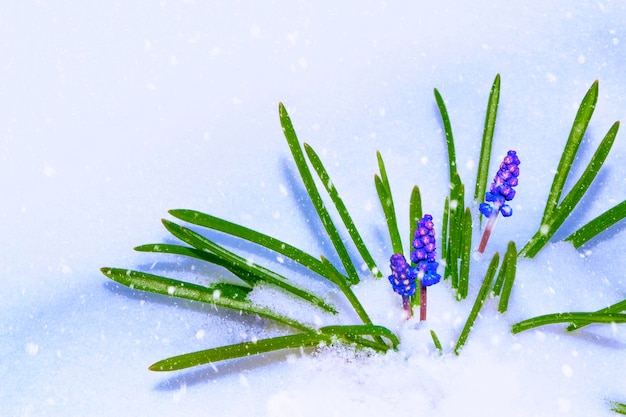The image depicts a computer-generated illustration of a plant emerging from a blanket of glistening, compact snow, covering approximately two-thirds to three-quarters of the frame. Little snowflakes can be seen falling between the viewer and the scene, adding to the wintry atmosphere. In the lower right-hand corner, a long-stemmed, grass-like plant spreads its green leaves in various directions. From this cluster of greenery, three reddish-brown stems rise, each crowned with tightly grouped, bulbous flowers in striking shades of purple and dark blue. The bright white snow, adorned with subtle blue shadows and sparkles, contrasts vividly with the vivid colors of the blooming flowers, creating a mesmerizing scene of nature's resilience.